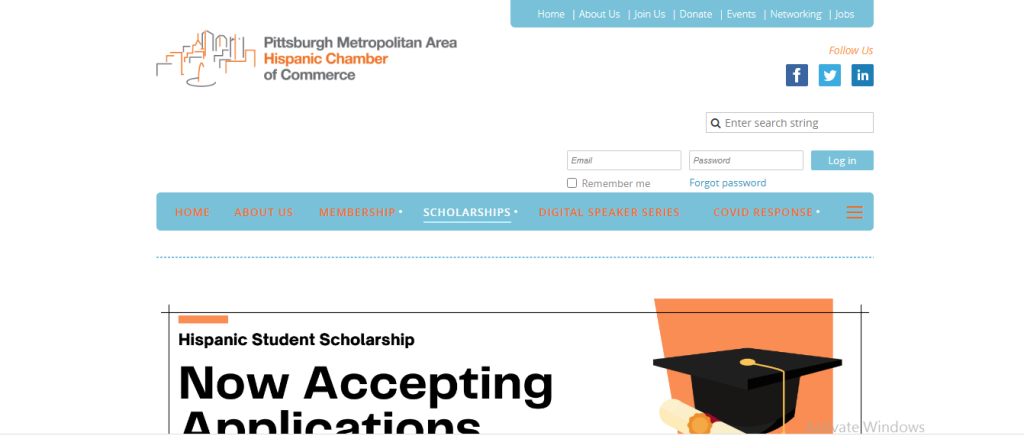The image is of a webpage from the Pittsburgh Metropolitan Area Hispanic Chamber of Commerce. At the top of the page are several navigational links including "Home," "About Us," "Join Us," "Donate," "Events," "Networking," and "Jobs." There are follow icons for social media platforms: a blue square with a white 'F' for Facebook, a blue square with a white bird for Twitter, and a blue square that may either represent Instagram or LinkedIn (indicated as 'IN'). 

Below these icons is a search bar, followed by text fields for "Email" and "Password," alongside a "Log In" button, a "Remember Me" checkbox, and a "Forgot Password" link. Further navigation includes links such as "Membership" (highlighted in orange), "Scholarships," "Digital Speaker Series," and "COVID Response" also in orange. A menu icon with three horizontal lines is present.

A prominent banner feature announces, "Hispanic Student Scholarship Now Accepting Applications" in black text. An orange square to the right showcases a detailed graphic of a black graduation cap with a gold tassel and a rolled-up diploma tied with a red ribbon secured with a gold seal.

At the very bottom of the image, there is a faint gray text that reads "Activate Windows."